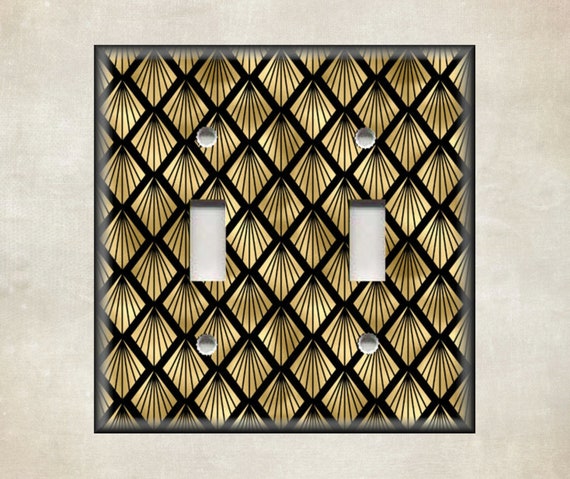The image depicts a double light switch plate cover lying on a beige background. The cover is square with space for two light switches, exhibiting a striking 1920s Art Deco design. A black border frames the plate, which is adorned with a repetitive pattern of gold fan-like shapes set within diamond configurations, creating a seashell appearance. The fan shapes face downward and are arranged in long rows, totaling about 50 to 60 individual fans. Additionally, there are small holes at the top and bottom of the plate for screws, and rectangular cutouts for the light switches themselves. The overall design is enhanced by the contrast between the detailed black grid and the intricate gold pattern, set against the neutral beige background.